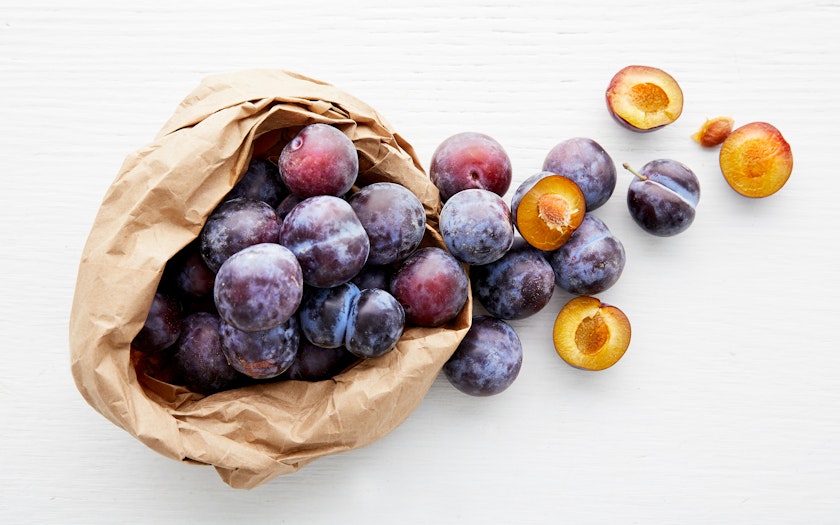This is a professionally composed photograph depicting a bounty of about 20 ripe and fresh plums placed on what appears to be a white painted wooden table. The scene is centered around a brown paper bag from which some of the plums are spilling out to the right. The plums are a rich purple color with a silvery sheen, indicating their freshness and high antioxidant content. Two of the plums have been sliced open, revealing their vibrant orange flesh and the stones inside. The lighting in the image is bright and natural, enhancing the rich colors and making it suitable for use in health magazines or blogs. There are no distracting elements like text or watermarks, allowing full focus on the fruit’s vivid details.